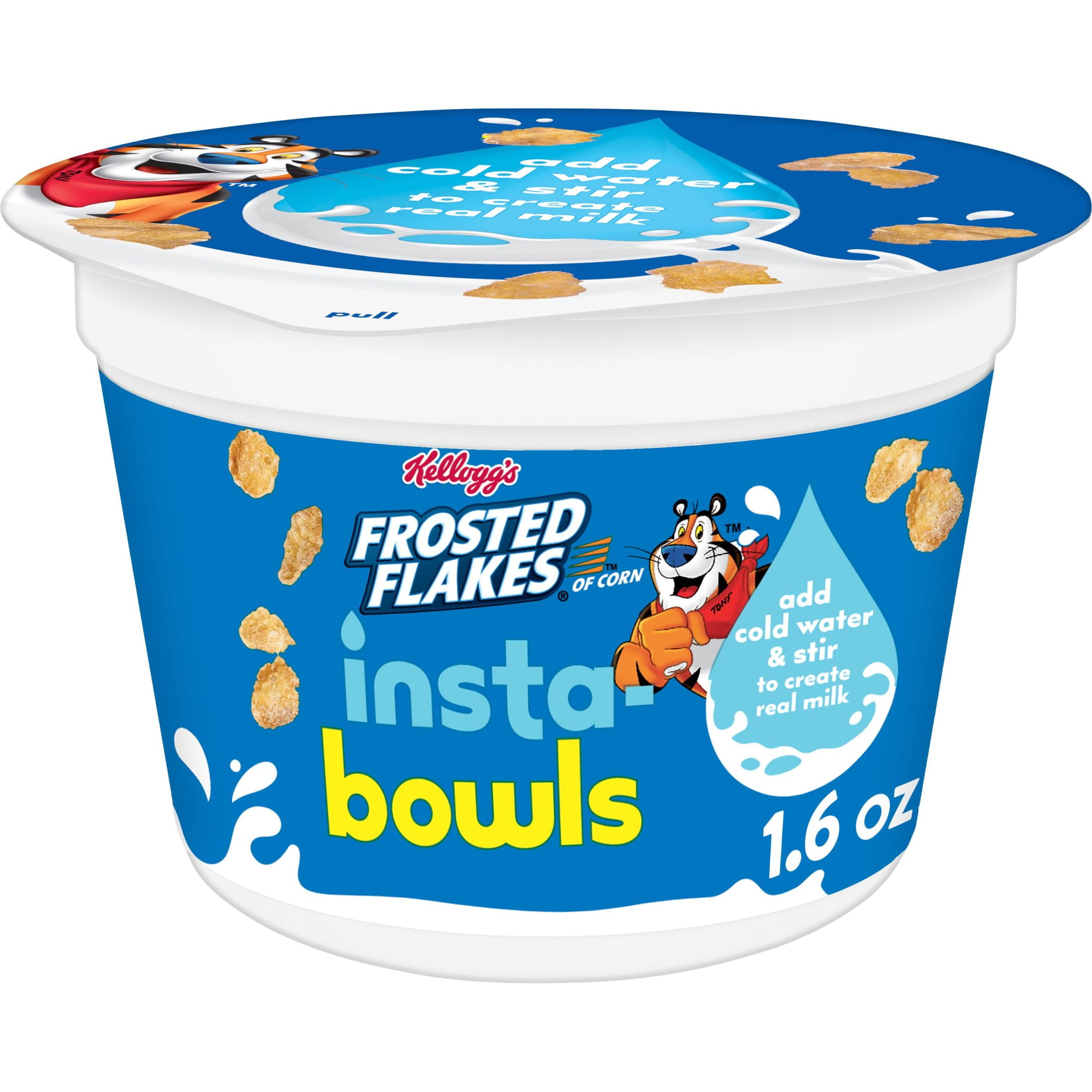This is a detailed product photograph featuring Kellogg's Frosted Flakes of Corn Instabowls. The image showcases a white plastic bowl with a navy blue pull-tab lid, labeled clearly with "Kellogg's Frosted Flakes of Corn Instabowls" in the center. The label design prominently features golden tan cornflakes falling from the top and splashes of white milk at the bottom. Near the top, the text "Kellogg's" appears in red cursive, while "INSTA" is written in light blue and "BOWLS" in yellow. The front also includes Tony the Tiger, sporting a red bandana, emerging from a light blue water droplet. Inside this droplet, it states in white text, "ADD COLD WATER AND STIR TO CREATE REAL MILK." The bowl has additional cornflakes and milk droplets scattered on both the lid and label. The entire product is encased in a navy blue wrap, highlighting the iconic Frosted Flakes branding, complete with Tony the Tiger's cheerful depiction and the product's weight, "1.6 OZ," displayed in white text.